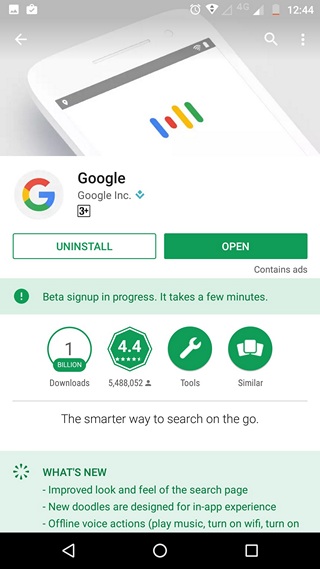Here is a clean and detailed caption for the image:

---

Screenshot of the Google Play Store installation page for the Google app. At the top, a generic visual representing Google is displayed. Below it, the Google app's logo is shown alongside the app name "Google" and the developer "Google Inc." The app is rated for ages 3 and up, indicated by a "3+" rating. 

Two prominent buttons are visible: a white "Uninstall" button with green text on the left, and a dark green "Open" button with white text on the right. Beneath these buttons, a green banner states "Beta sign up in progress," noting that the process takes a few minutes. 

Further down, the app's credentials are listed: it has been downloaded over 1 billion times, holds a rating of 4.4 out of 5 stars from 5,488,052 reviews, and falls under the category "Tools." Additionally, there are options to explore similar apps. 

At the bottom of the page, a section highlights recent updates made to the app.